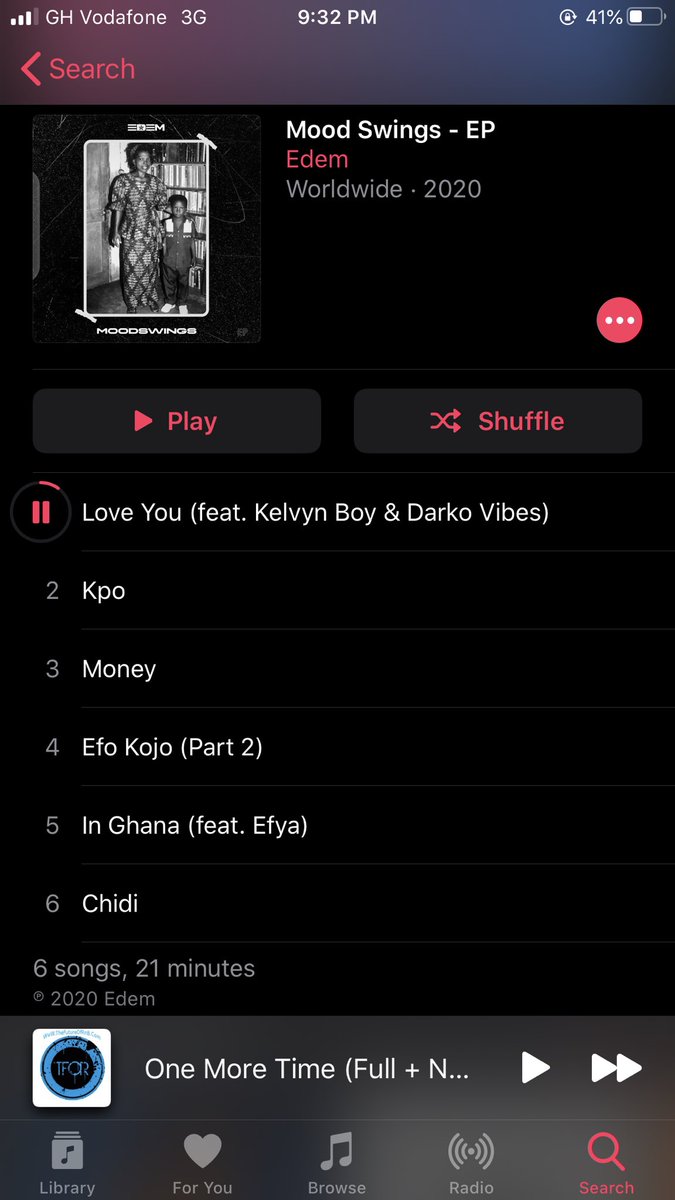A detailed phone screenshot of a music app interface:

**Top Section:**
- **Background:** Bluish-black.
- **Header Text (in white):** Displays cellular indicators (signal strength, "GH Vodafone 3G"), and the current time (9:32 PM).
- **Icons:** A refresh button with "41%" indicating battery percentage, alongside a battery icon showing it is more than half drained.

**Middle Section:**
- **Navigation:** On the left, a red back arrow and search icon.
- **Album Art:** Displaying a black and white photo of what appears to be a mother and child.
- **Album Info:**
  - **Title (in white):** "Mood Swings EP"
  - **Artist (in red):** "Eat Em"
  - **Release Info (in gray):** "Worldwide 2020"

**Below the Album Art:**
- **Control Buttons:** A play button and a shuffle button.
- **Current Song:** A red-progress circle indicating partially played song.

**Track List (in white, indicating active or current status):**
1. "Love You"
2. "K-Po"
3. "Money"
4. "Ifo Kofo, Part 2"
5. "In Ghana"
6. "Shitty"

**Additional Information:**
- **Album Length (in gray):** "6 songs, 21 minutes"
- Bottom Navigation (in gray): Options for "Library," "For You," "Browse," "Radio," and "Search."

This detailed description offers a comprehensive view of the music app interface shown in the screenshot, highlighting its design, functionality, and content effectively.